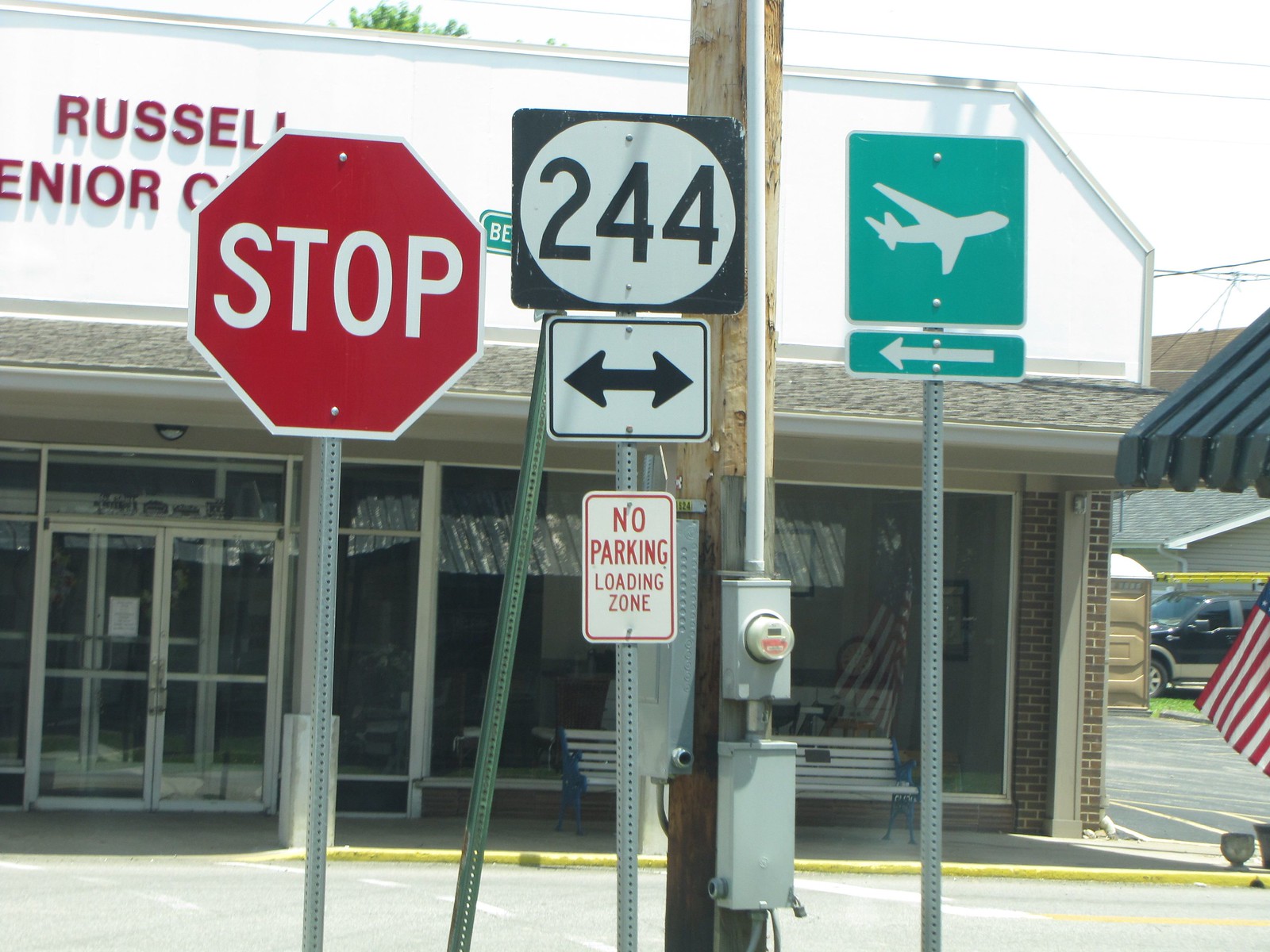This outdoor photograph captures a bustling street scene with multiple street signs and a large storefront in the background. Dominating the foreground are several poles with various signs: a prominent red stop sign on a dark gray pole, a rectangular green street sign partially obscured, and a route marker labeled "244" in black text on a white circle with an arrow beneath it indicating both directions. Below this is a smaller sign reading "NO PARKING LOADING ZONE" in red text. Additionally, there is a green sign with a silhouette of an airplane and a left-pointing arrow. Behind these, the storefront spans a large section of the image, featuring numerous windows filled with indiscernible items. The store's signage reads "R-U-S-S-E-L" and is partially obscured by the stop sign, followed by the letters "E-N-I-O-R" suggesting the word "Senior," and culminates in a partially visible 'C'. The lettering is red with a white and light gray painted shadow effect. The entrance boasts glass double doors framed in silver. To the front right, an American flag is visible, and there is also a tan porta-potty on the edge of a parking lot. The parking lot itself is a mix of dark and light gray asphalt, marked with yellow lines and showing signs of aging through visible cracks. Two concrete barriers mark parking spaces. A black truck and a tan building with a gray roof and white spouting are visible in the distance. The scene is bright and sunny, casting varying shades of gray on the sidewalk, which is particularly light where the sun hits. Peeking from behind the building is part of a tree, adding a touch of greenery to this detailed urban snapshot.